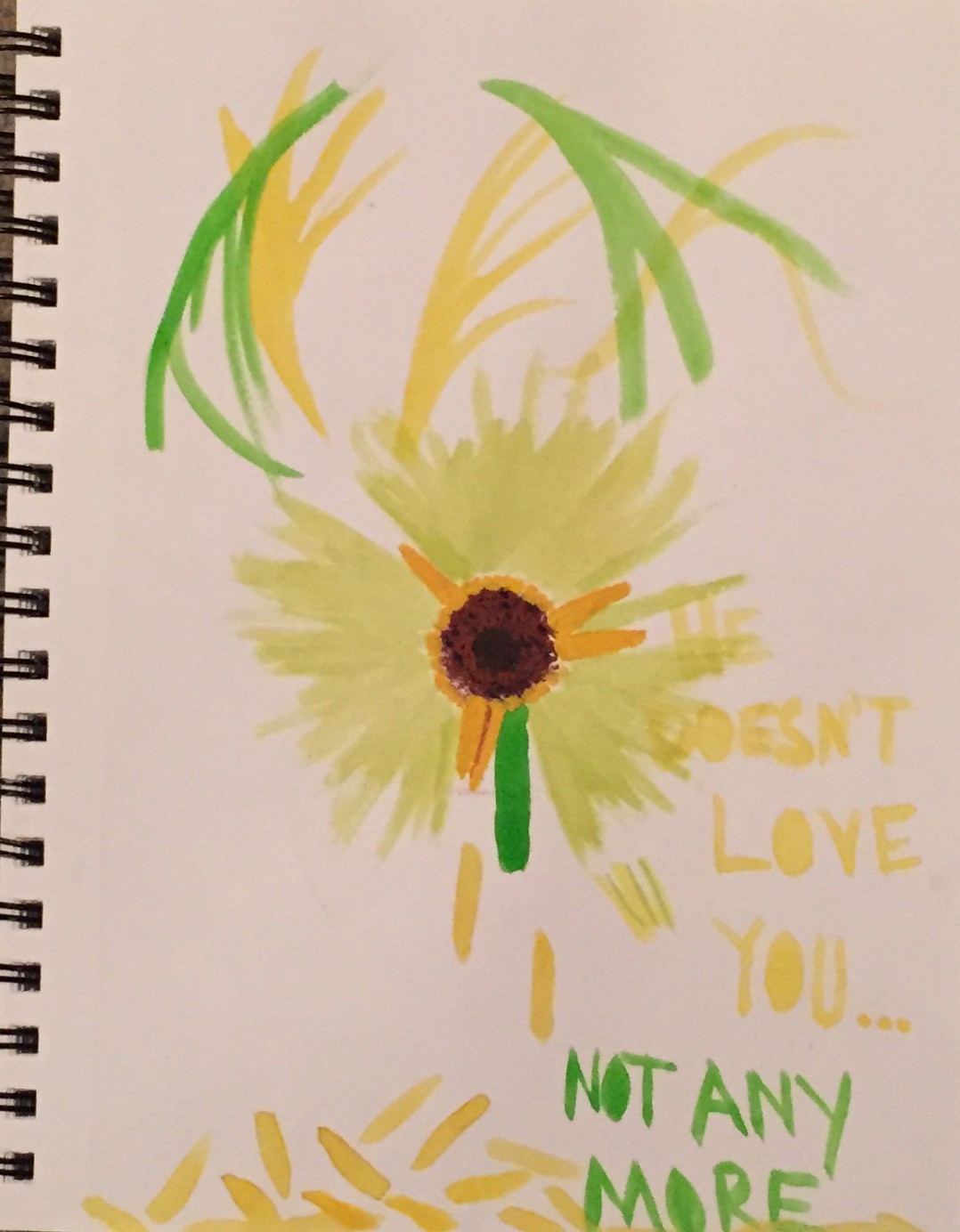This image captures a watercolor-like painting on a light lavender sheet from a spiral-bound drawing pad, slightly visible on the left side. The painting, which might be of a pansy, features a flower with a dark brown and black center surrounded by orange-yellow and green petals. Yellow shootouts extend from various points of the flower, with one at the top left, one from the bottom, and two from the right. Scattered yellow petals fall from the flower, accumulating in a pile below. A dark green stripe runs down from the middle of the flower, merging into the predominantly yellowish-green petals. Additional yellow and green lines and elements are featured around the flower, creating a dynamic composition. On the right side of the painting, text in yellow reads, "He doesn't love you...", followed by "not anymore" in green beneath it.